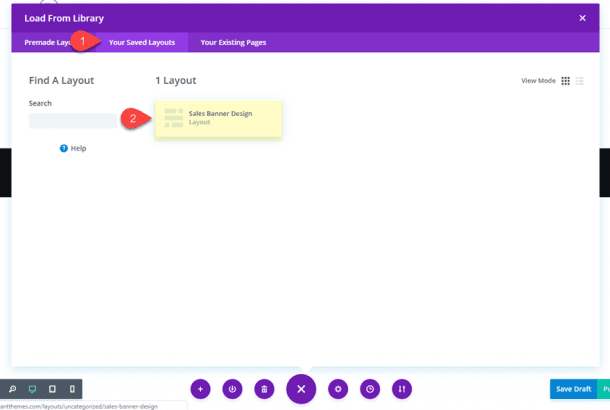**Detailed Caption:**

This screenshot captures a segment of a web application interface designed for layout management. Dominating the top portion of the interface is a conspicuous purple bar stretching across the screen. On the top left corner of this purple bar, bold white text reads "Load from Library," while on the top right corner, a white 'X' icon indicates the option to close the window.

Partially visible behind this window is the upper part of an unidentified icon, hinting at an underlying layer of the application. Directly below the "Load from Library" text are three menu choices, also set against a purple background. The first menu option is partially obscured and reads "Pre-made Lay..." with only the letters "L-A-Y" clearly visible. An orange, circular icon with the number '1' superimposes on this menu option, likely indicating relevance or priority.

The second menu choice, highlighted in a lighter shade of purple and drawing attention from the orange icon with the number '1', reads "Your Saved Layouts." The third option, listed as "Your Existing Pages," completes the menu selections.

Beneath these menu bars, the background switches to a clean, mostly white design. Prominently, it displays a header saying "Find a Layout." A search bar resides directly below this heading, presently empty. Adjacent to the search bar is a small, blue question mark icon labeled "Help," offering user assistance.

To the right of this help icon, the text "1 Layout" appears, accompanied by another orange icon displaying the number '2'. This icon directs attention to a yellow-bordered box labeled "Sales Banner Design Layout." 

On the far right of the interface, near the top, "View Mode" is indicated with a currently active icon representing a 3x3 grid of dots. Next to this grid icon, in a grayed-out state, is another icon resembling bullet points accompanied by lines, suggesting a list view mode.

The detailed structural elements and thoughtful use of color and icons collectively enhance the user experience by providing clear navigation and intuitive control within the web application.